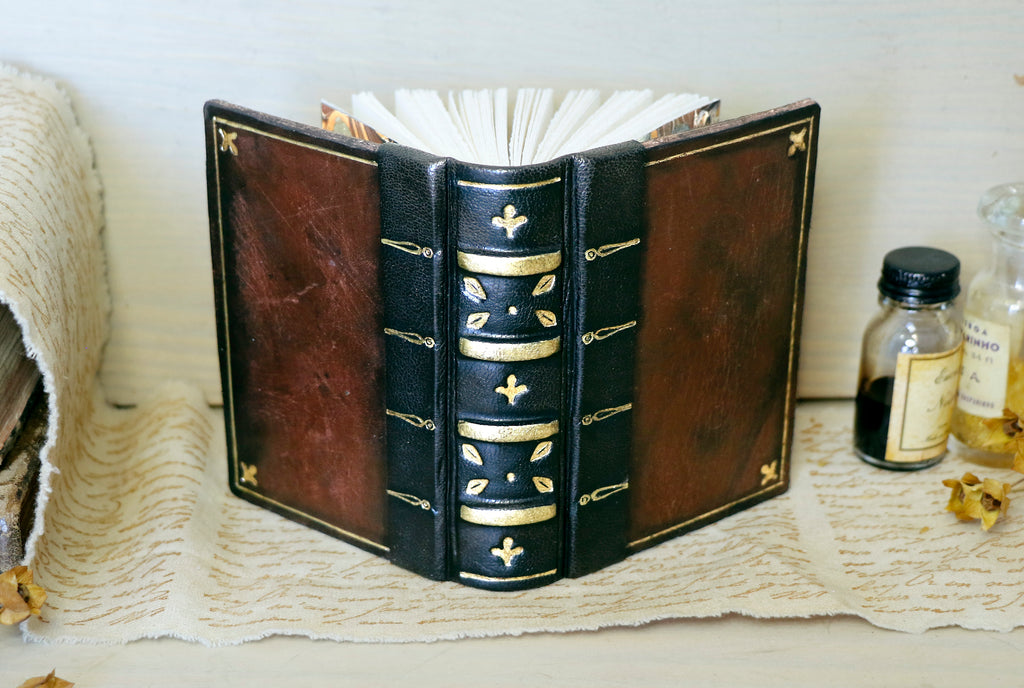In this colored indoor photograph, a vintage leather-bound book is prominently displayed atop a white shelf. The shelf backs onto a matching white wall. The book, which has a brown leather cover with intricate gold foil decorations and a black leather spine, is fanned open with its spine facing the viewer, revealing cream-colored pages and full-page illustrations on the inside covers. Both the front and back covers are adorned with gold edging and decorative cross markings in the corners. 

The book rests on an elegantly draped cloth, which flows down over a table. This cloth features handwritten, cursive text in a yellowish or goldish color. Flanking the book are two small bottles with aged, discolored labels; one contains black liquid, and the other holds an orange gel. Additionally, a couple of dried flowers lie nearby, enhancing the vintage, scholarly ambiance of the scene.